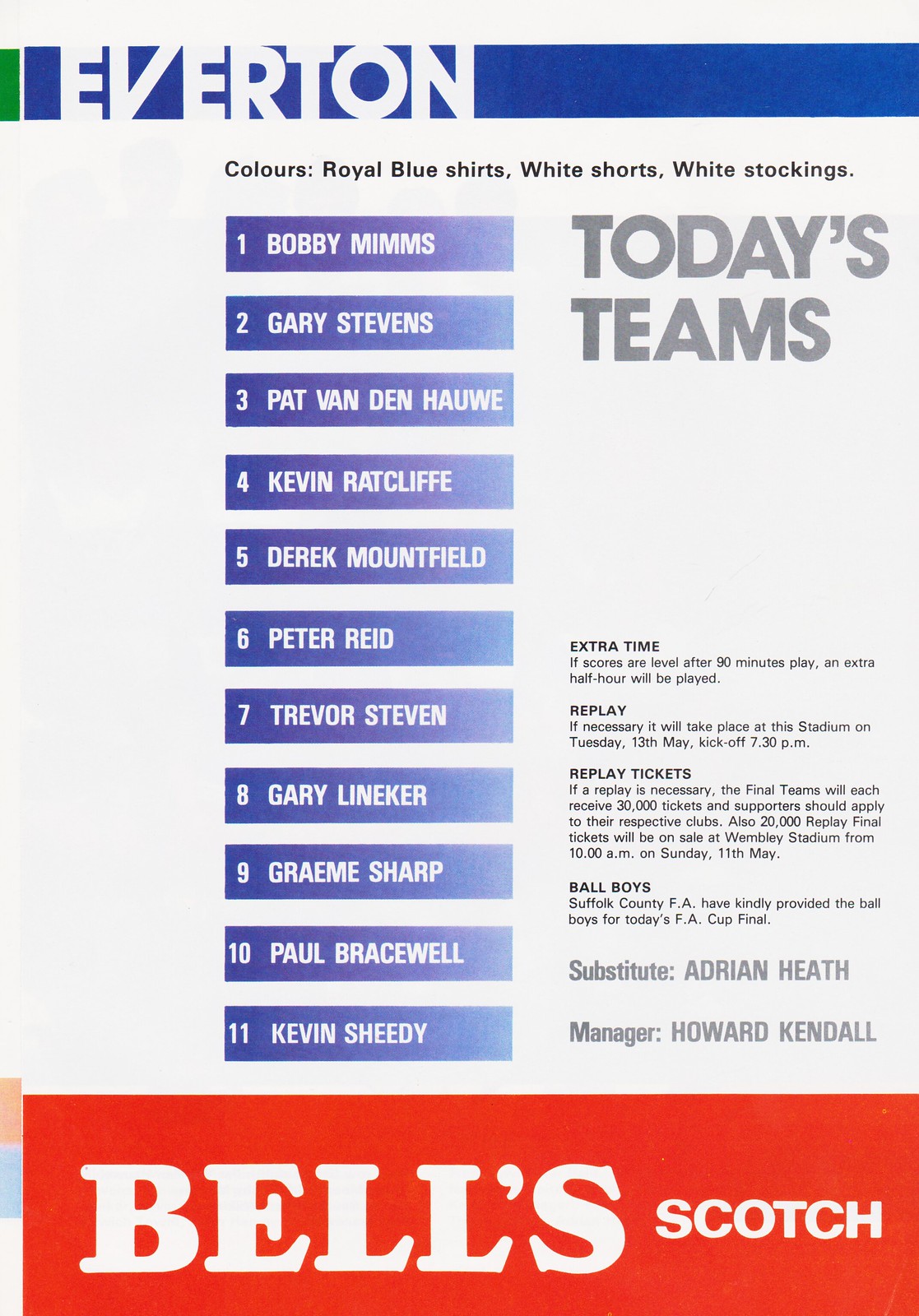This detailed sports team lineup page, likely from a magazine, prominently features the Everton team for the day. At the very top, a horizontal blue bar emblazoned with "EVERTON" in large white capital letters stretches across the page. Directly below, it lists "Colors: Royal Blue Shirts, White Shorts, White Stockings" in black text against a light gray backdrop. The central content is dominated by a vertical list of players numbered 1 to 11, each name encased within a blue box with white text, beginning with Bobby Mims at number 1 and concluding with Kevin Sheedy at number 11. To the right, in capital light gray letters, the section reads "TODAY'S TEAMS." Further down, black text provides detailed information about Extra Time, Replay, Replay Tickets, and Ball Boys. Additionally, it mentions the substitute, Adrian Heath, and the manager, Howard Kendall, in gray letters. The page wraps up with a red banner at the bottom, displaying "BELL'S SCOTCH" in bold white letters, resembling an advertisement. The overall color scheme balances blue, red, light gray, and white, with splashes of black and gray text, creating a vibrant yet organized presentation.